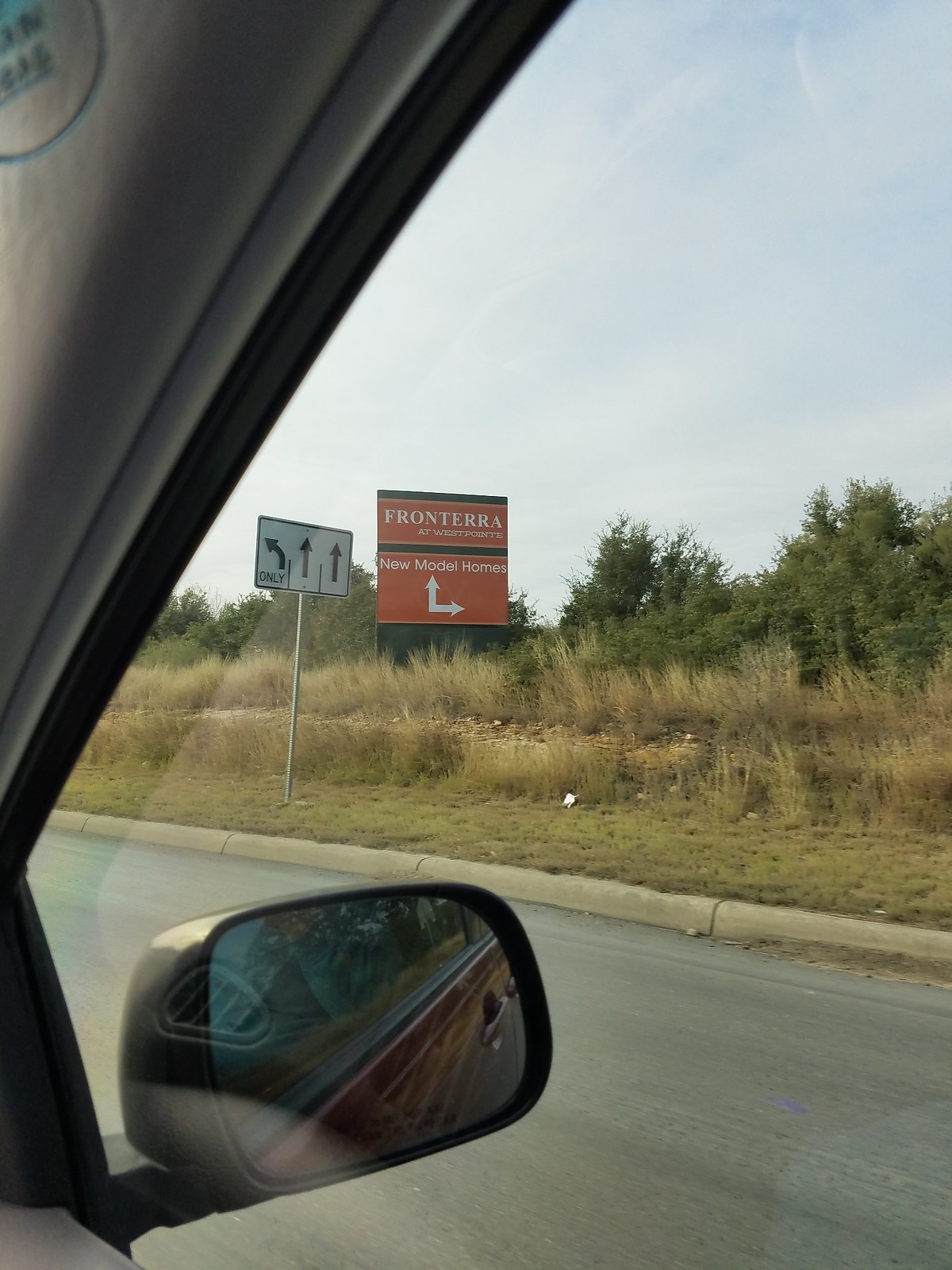Captured from the interior of a vehicle, possibly a car or truck, this photograph presents a detailed view through the window, which is framed by a hint of gray trim. The vehicle's dark red exterior is subtly reflected in the visible side mirror. The scene outside reveals a street bordered by a cement curb, leading to a stretch of grass. Beyond the neatly manicured grass, the landscape transitions into a wilder, overgrown area teeming with weeds, bushes, and various wild plants. Dominating the scene is a red sign that reads "Frontier at West Point," directing potential buyers to new model homes with prominently displayed arrows.